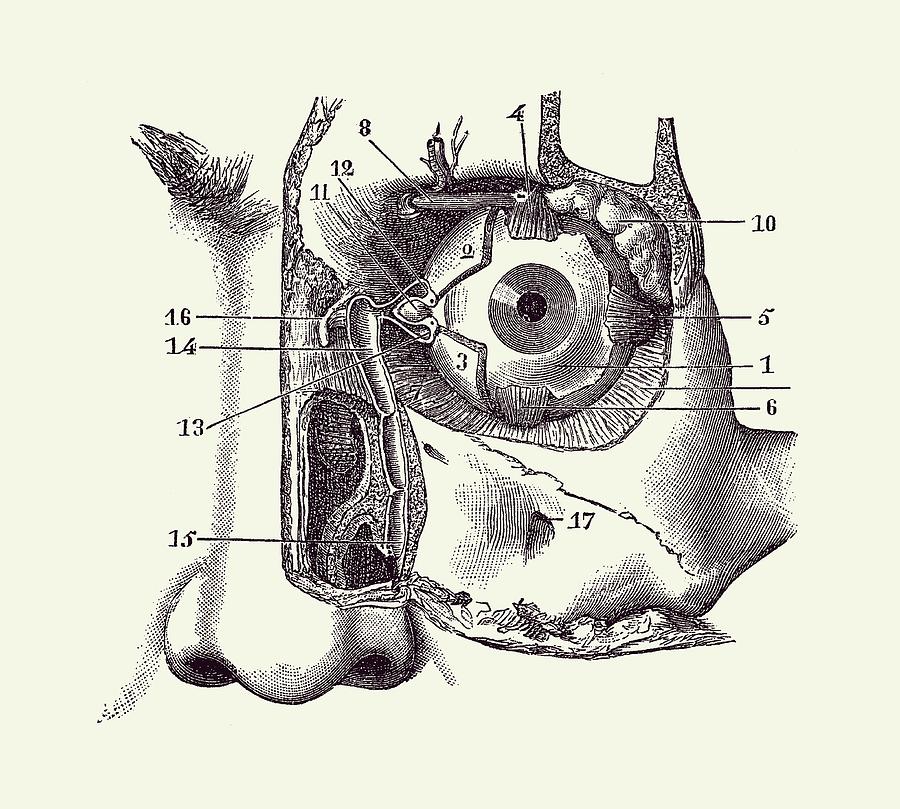This black-and-white pen and ink drawing is a detailed anatomical diagram of the face, focusing primarily on the eye and surrounding orbital area. It features a partially peeled-back view of the skin, revealing the muscles, nasal cavity, and cheekbone beneath. The eye is prominently displayed without its eyelids, exposing the pupil, iris, and associated muscles, while the surrounding areas, including the nose and eyebrow, are meticulously numbered from 1 to 17. Arrows point to different parts of the anatomy, making it explicit which sections are being highlighted. The style suggests it may have originated from an older medical textbook or a doctor's office from a previous era, aimed at providing a scientific view of human facial anatomy.